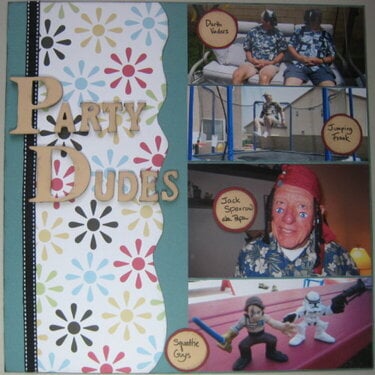The photograph depicts a detailed and colorful scrapbook, prominently displaying a blue spiral-bound cover. A white strip adorned with multicolored starbursts—black, red, yellow, and green—embellishes the cover. "PARTY DUDES" is inscribed in gold capital letters across this strip. The scrapbook's format is almost square, slightly elongated lengthwise. The right side presents a column of four distinct photographs: the top image features two people sitting on a sofa, followed by a man bouncing on a trampoline, beneath that a man in a red fez hat and a flowered blue shirt with markings under his eyes, and at the bottom, two toy figures—one grasping a blue lightsaber and the other resembling a Star Wars stormtrooper with a large black gun. Each photo is labeled with tan circles outlined in red, containing handwritten black annotations. The left side, contrastingly, showcases a single large image, covered partly by material displaying a colorful floral pattern.